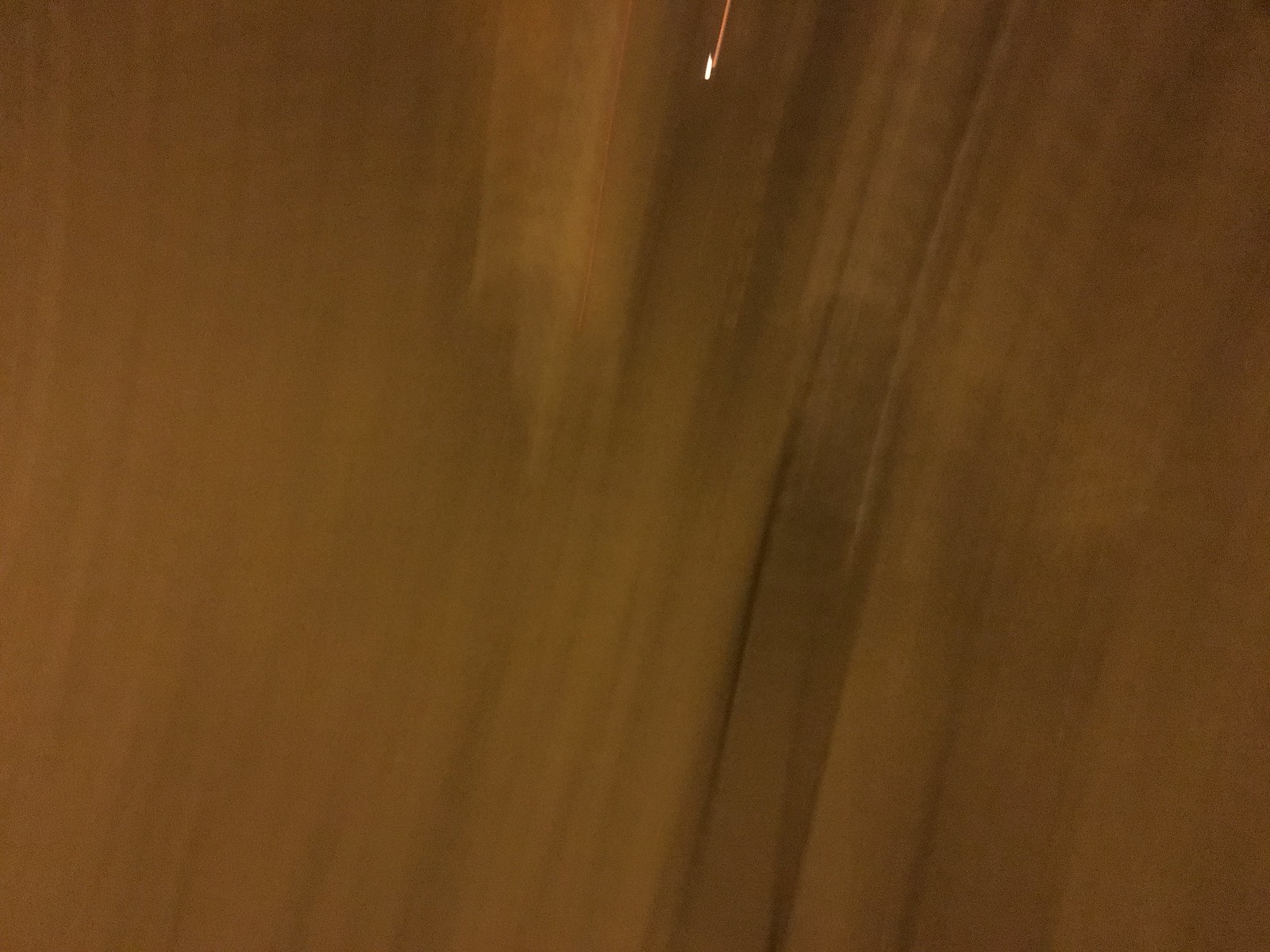This image captures a close-up of a medium-toned wooden surface with a reddish background. The open, smooth wood grain adds texture and movement, transitioning from a more pronounced grain pattern on the left to a smoother surface on the right. The color palette spans from light umber to a rich, dark oak, creating visual depth and warmth. Near the top center, a small white dot—approximately a quarter of an inch wide—stands out, accompanied by a thin red line extending above it, adding a subtle focal point to the composition.